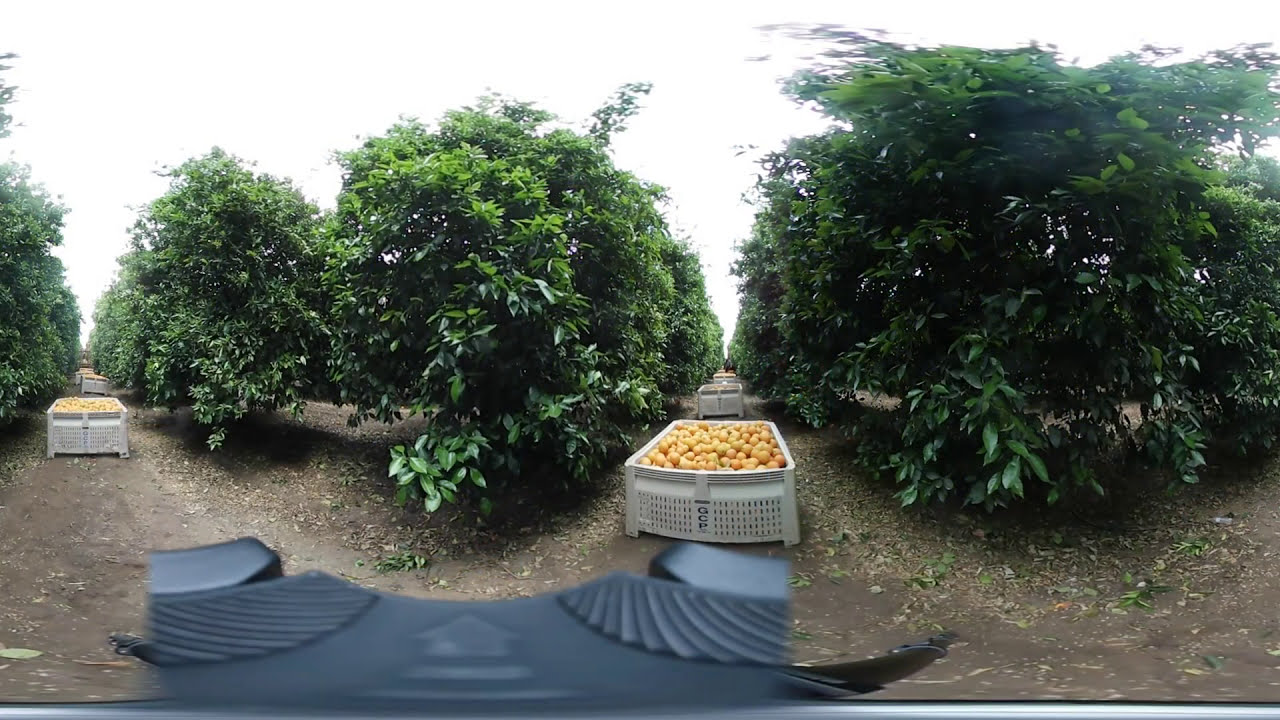The image depicts a panoramic view of a fruit-picking area on a cloudy day characterized by white overcast skies. Dominating the scene are numerous rows of orange trees with sizable green leaves, though no fruit is visible on the plants. Between these rows, sandy lanes in a slightly dark brown and blackish color extend, lined with fallen leaves. Scattered along the lanes are large, whitish-grey plastic containers filled to the brim with oranges, each likely housing hundreds of them. Prominently displayed on the side of one central container are the letters "GCP." A total of five such containers filled with oranges are spread out along the view, with three or four positioned towards the back. At the bottom edge of the image, a portion of a black vehicle is visible, offering a vantage point from where the scene is being observed.